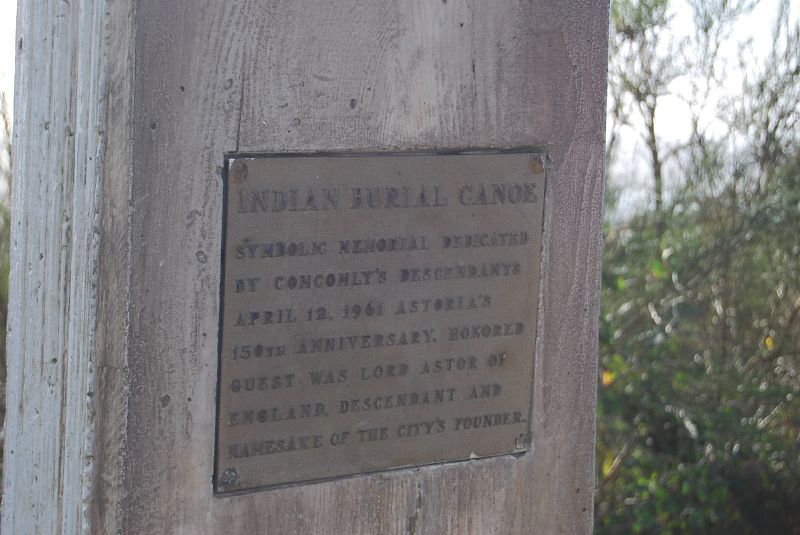The image depicts an outdoor setting taken during the daytime. On the left-hand side of the photograph, there is a weathered wooden structure, potentially representing the bottom of a canoe, painted in a grayish-brown hue. Mounted on the front of this structure is a square metal plaque, fastened with bolts at each corner. The plaque is bronze with black raised print and reads: "Indian Burial Canoe. Symbolic memorial dedicated by Kinkali's descendants. April 12, 1961, Astoria's 105th anniversary. Honored guest was Lord Astor of England, descendant and namesake of the city's founder."

The background features a green bush at the bottom and a relatively gray sky, with a few trees and brush visible. This setting creates a somber yet respectful atmosphere, emphasizing the historical significance of the memorial site.